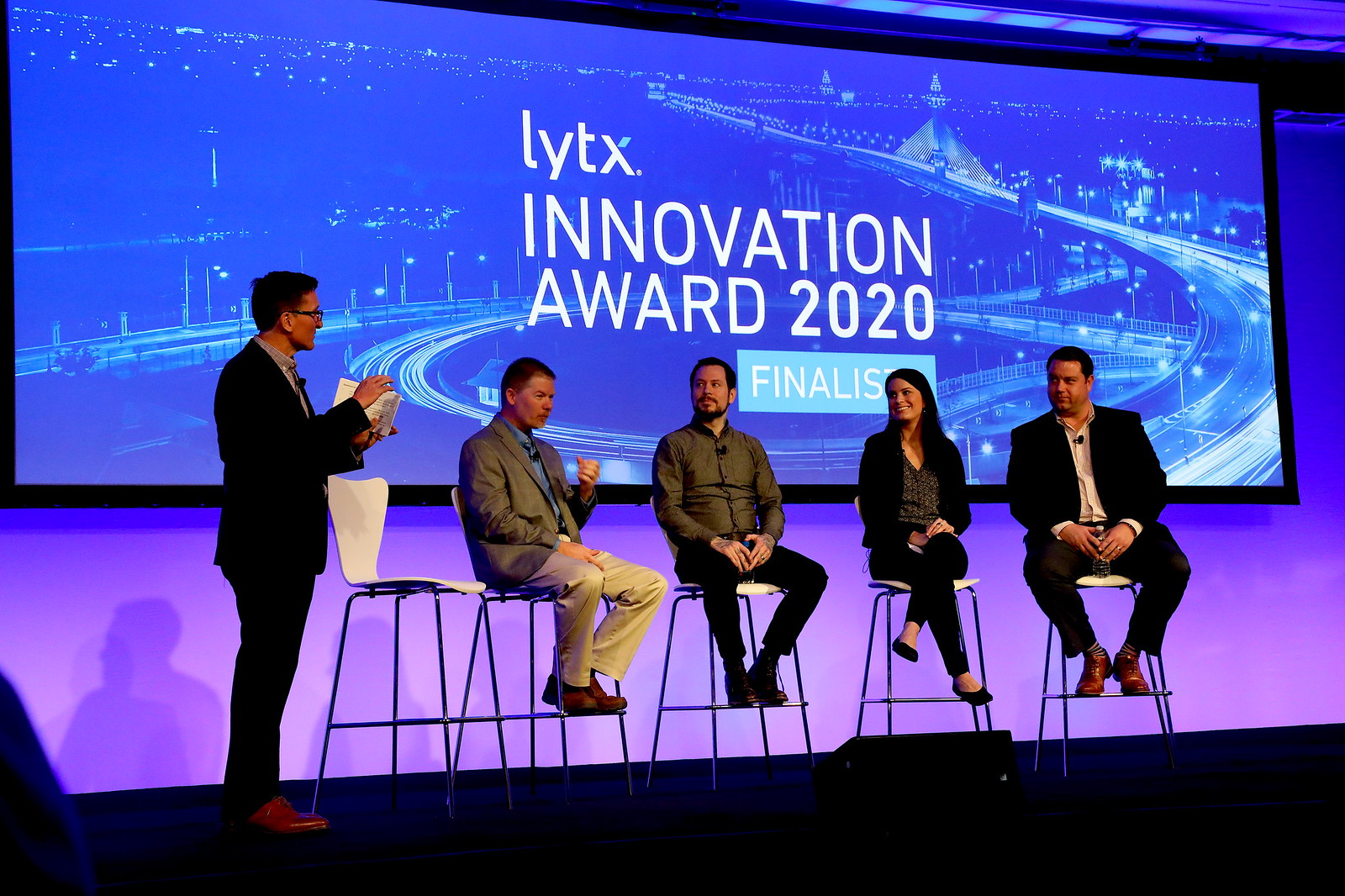This indoor photograph captures a stage setup featuring five high, white chairs with blue metallic legs. Four individuals are seated, comprised of three men and one woman, all of whom are white. To the left, a man, also white with dark brown hair, glasses, a dark suit, and brown shoes, stands by the empty chair. He holds a piece of paper and appears to be addressing the seated group. Behind them is a large display screen with an aerial view of a city and the text "LYTX Innovation Award 2020 Finalists." The scene suggests an ongoing introduction or announcement related to the award, with everyone's attention focused on the standing man.